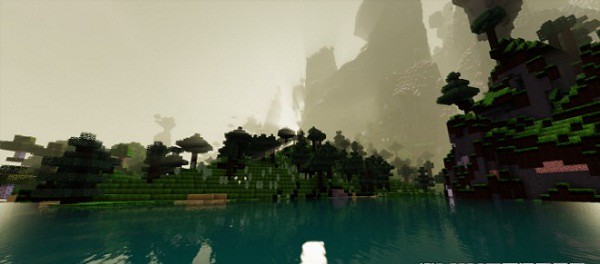The image appears to be a scene from a video game with a modular, blocky design reminiscent of Minecraft. At the bottom of the picture, there is a body of water. To the right, there is an island primarily depicted in black, featuring several green steps and possibly some trees. Straight ahead lies another island that is more vibrant with greenery and trees, dotted with some buildings. The sky above is gray, adding a foggy, atmospheric quality to the scene. In the background to the right, there are large structures, potentially castles, which appear blurry and faded due to the foggy conditions.